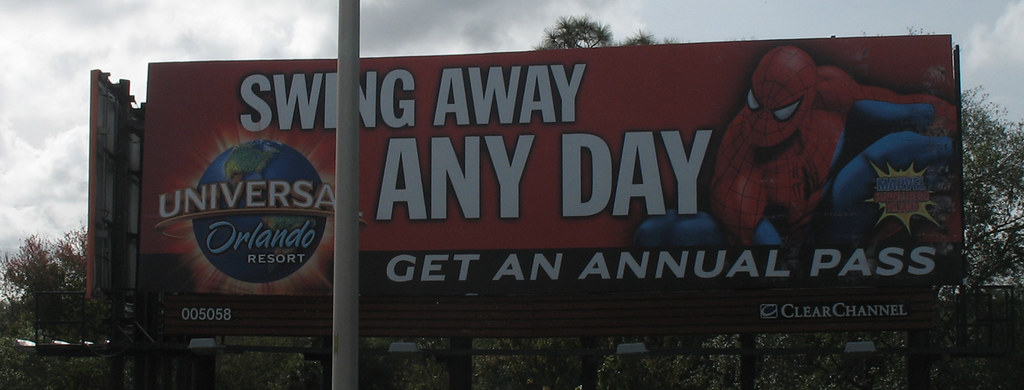A highly detailed roadside billboard promoting a Spider-Man attraction dominates the image. The billboard features a vibrant depiction of Spider-Man on the right side, poised in an action-ready stance. To the left, bold white capital letters proclaim "SWING AWAY," followed by an even larger "ANY DAY." Beneath this, the message "GET AN ANNUAL PASS" suggests a promotional offer, possibly for a new Spider-Man ride at Universal Orlando Resort. This text is emblazoned across a globe, symbolizing the Earth, reinforcing the global allure of the attraction. The left-most section of the billboard features the Universal Orlando Resort logo. In the bottom right corner, the name "Clear Channel" indicates the advertising company. In the background, lush trees frame the scene, while a white pole stands visibly in front of the billboard, adding depth to the composition.